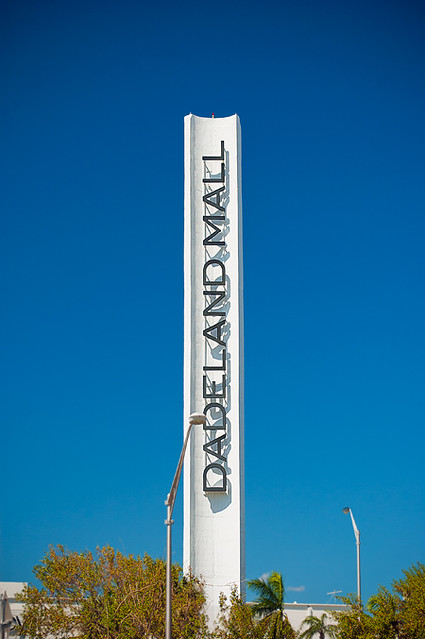This image captures a tall, vertical sign for Dadeland Mall, prominently displayed against a clear, cloudless blue sky. The sign, an elongated white pillar with concave curved edges, features the words "Dadeland Mall" in large, black capital letters arranged vertically. This towering structure stands much taller than the nearby streetlights, one of which is positioned directly in front of the sign and reaches up to around the "D-A-D" portion of the text. At the base of the sign, green foliage and palm trees suggest a tropical location, likely Miami-Dade County, enhancing the summery atmosphere of the scene. A white flat building is visible at the bottom, partially obscured by the lush greenery. The overall setting hints at a bright, sunny day, presumably in the afternoon, with two streetlights poised to illuminate the area after sunset.